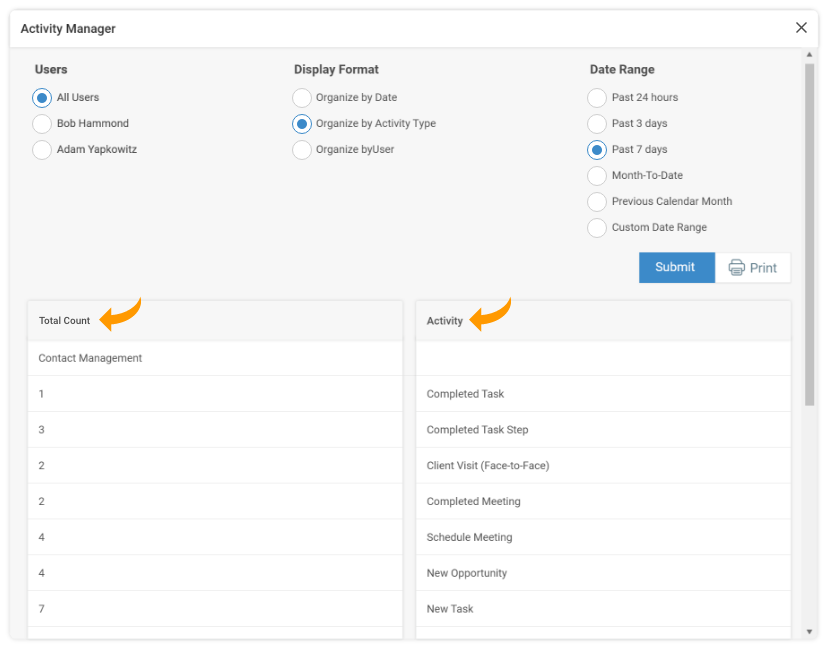A detailed screen capture displays the interface of an activity manager application on a computer or tablet. The square-shaped image features a light gray, almost white, background with a dark gray scroll bar on the right side, positioned at the top. In the upper left corner, the page is labeled as the activity manager. The upper right corner includes an "X" icon to close the application.

The application pop-up at the top contains three columns. The left column, labeled "Users," includes options for "All Users," "Bob Hammond," and "Adam Japsiewicz," with "All Users" highlighted in a blue bubble. The middle column, "Display Format," offers choices organized by date, activity type (selected and highlighted in a blue bubble), and user. The right column, "Date Range," presents options for the past 24 hours, past three days, past seven days (selected), month-to-date, previous calendar month, and a custom date range. Below these options, a blue "Submit" button and a white "Print" button are visible.

At the bottom of the page, there are two white squares. The left square, titled "Total Count," is marked by an orange curved arrow and contains a section labeled "Contact Management" with the numbers one through seven listed vertically. The right square, named "Activity," features a similar orange arrow pointing to it and lists activities such as "Completed Task," "Completed Task Step," "Client Visit Face-to-Face," "Completed Meeting," "Scheduled Meeting," "New Opportunity," and "New Task."